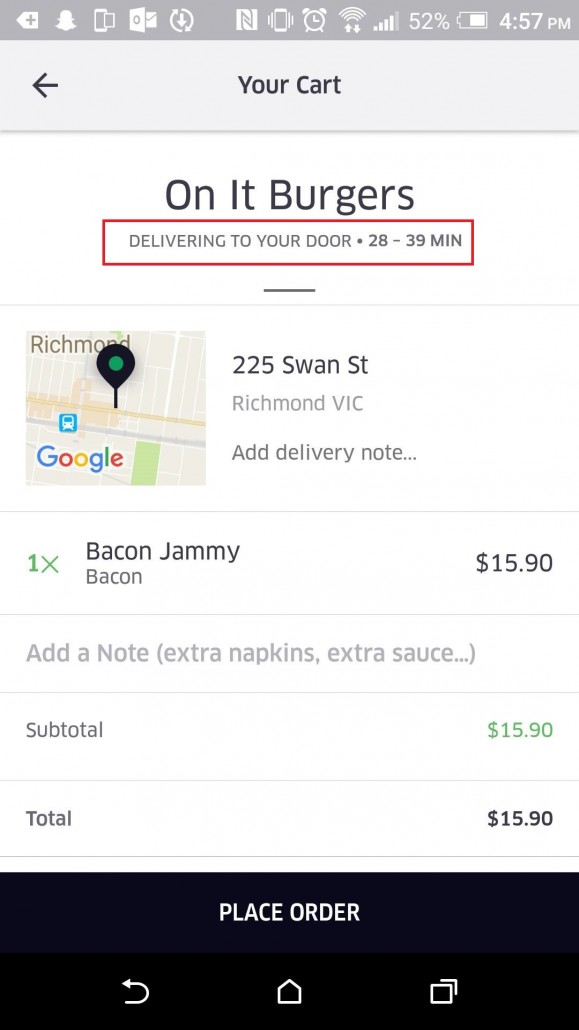Screenshot taken at 4:57 PM with a battery level of 52%, displaying an app interface for ordering food. An alarm clock symbol is present, indicating the delivery status. The section titled "Your Cart" features a left-pointing arrow, suggesting navigation capabilities. The app promises burger delivery within 28 to 39 minutes. The delivery heading is highlighted in a red rectangle beside a map pinpointing the delivery address in Richmond, specifically 2-5 Swan Street, Richmond, Victoria (Vic). A delivery note section includes an order for "1x Bacon Jammy" priced at $15.90, with options to add a note for extra napkins, extra sauce, etc. The subtotal and total amounts are both $15.90. There is a "Place Order" button, accompanied by a refresh symbol, a home icon, and two squares likely representing recent activity or additional menu options.